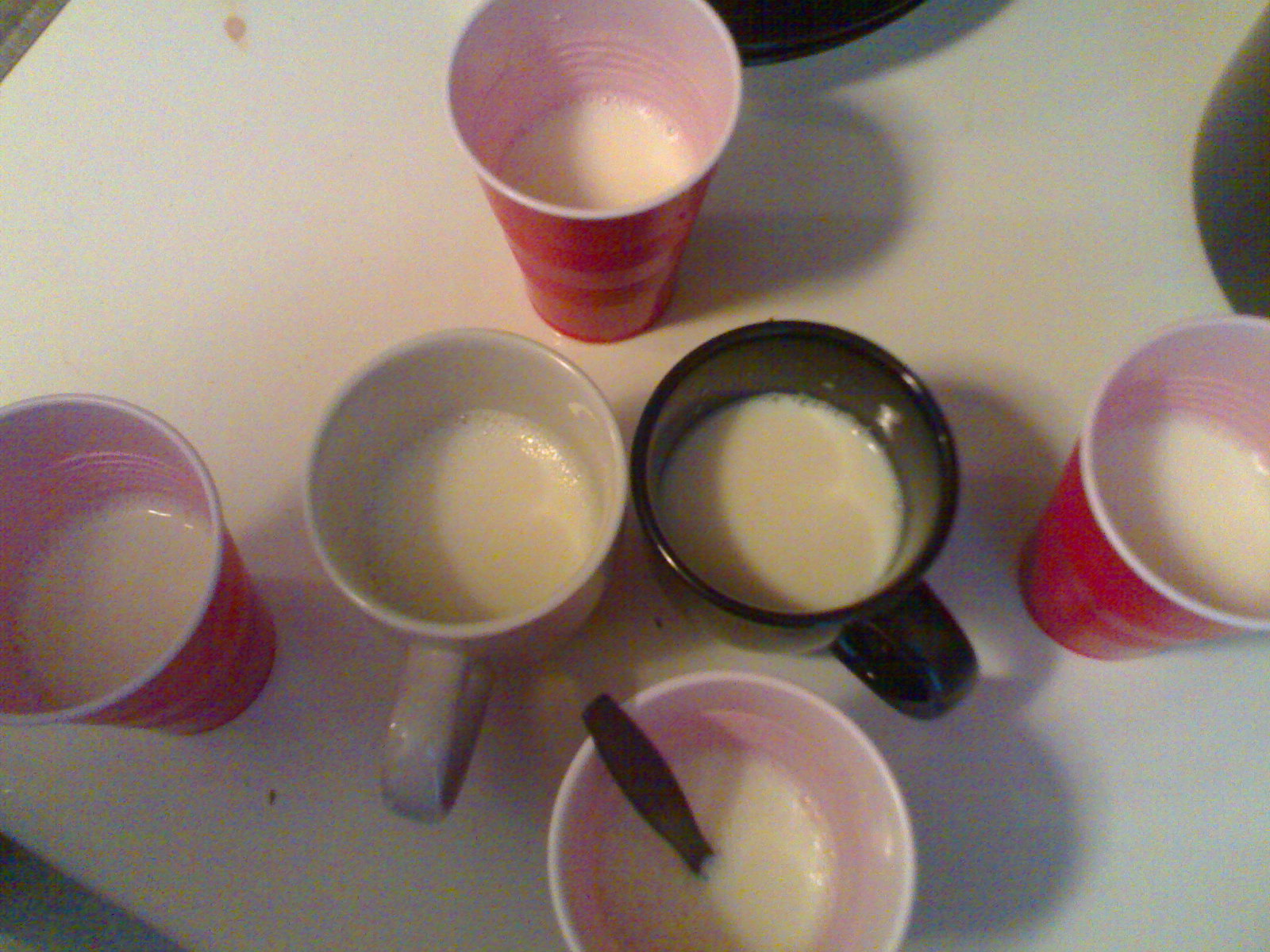The image is a color photograph displayed in landscape orientation, capturing a white countertop illuminated by overhead light, creating distinct shadows. The scene features six cups arranged on the table. This includes four red Solo plastic cups, each filled between halfway and two-thirds full with a milky white liquid. One of these cups, positioned at the bottom center, has a black plastic spoon protruding from it. Additionally, there's a white ceramic mug to the left and a black ceramic mug to the right, both also containing the milky substance. The photograph is taken from an elevated angle, providing a clear view into the cups and revealing their contents. At the top of the image, partially obscured, are two more black objects—likely another mug and potentially a black plate—adding to the complexity of shadows on the countertop. The image has a slightly grainy texture, with some red and black stains visible on the surface of the table.